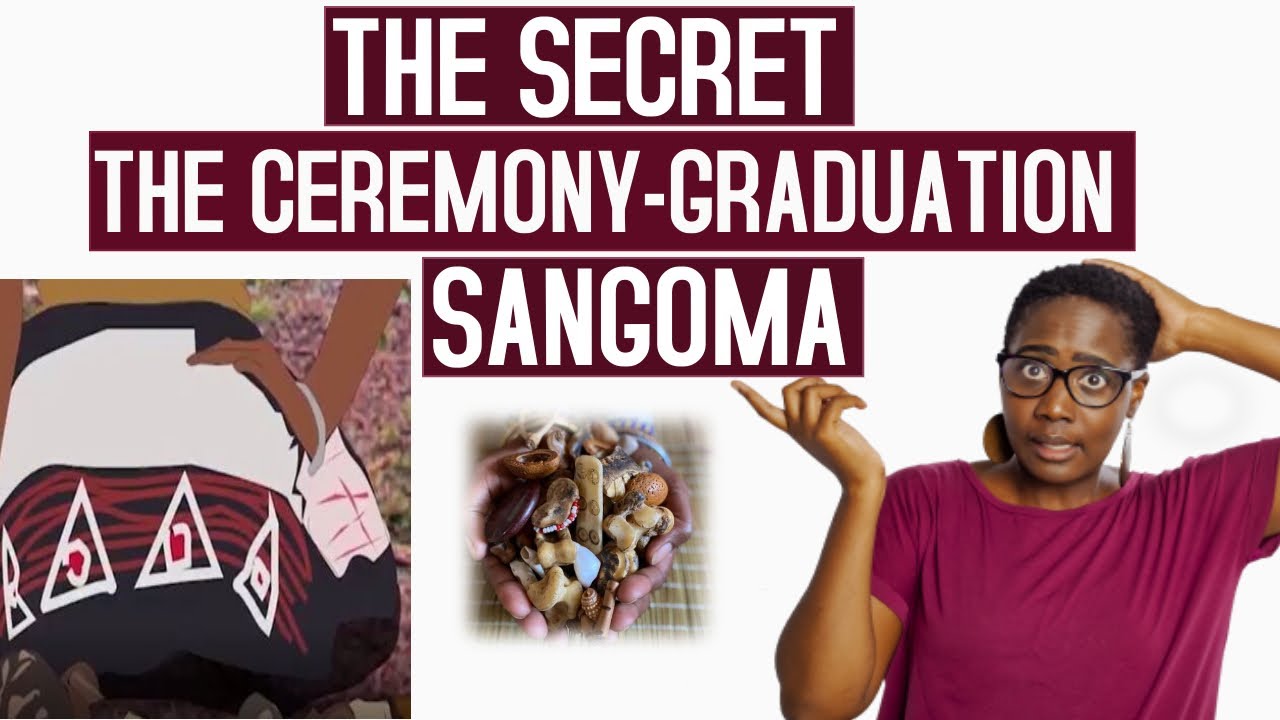This banner, which appears to be for a blog or how-to guide, features a clean, predominantly white background with three distinct red rectangles containing bold white text. The top red rectangle reads "The Secret," the middle reads "The Ceremony Graduation," and the bottom reads "Sangoma." Below the text, there are three photographs positioned on the white background. 

On the left is a 3D rendition of a woman draped in a decorative blanket skirt, characterized by a white and black pattern with red lines and white triangles. In the center is an image showcasing a person holding several rocks or similar items in their hands. The photograph on the bottom right features a younger African-American woman with short black hair and eyeglasses. She is wearing large, round earrings and a short-sleeved red shirt, with one hand behind her head and the other pointing upwards as if in emphasis or curiosity. The cohesive design and detailed imagery of the banner effectively draw the viewer's attention to the intriguing text and visuals.